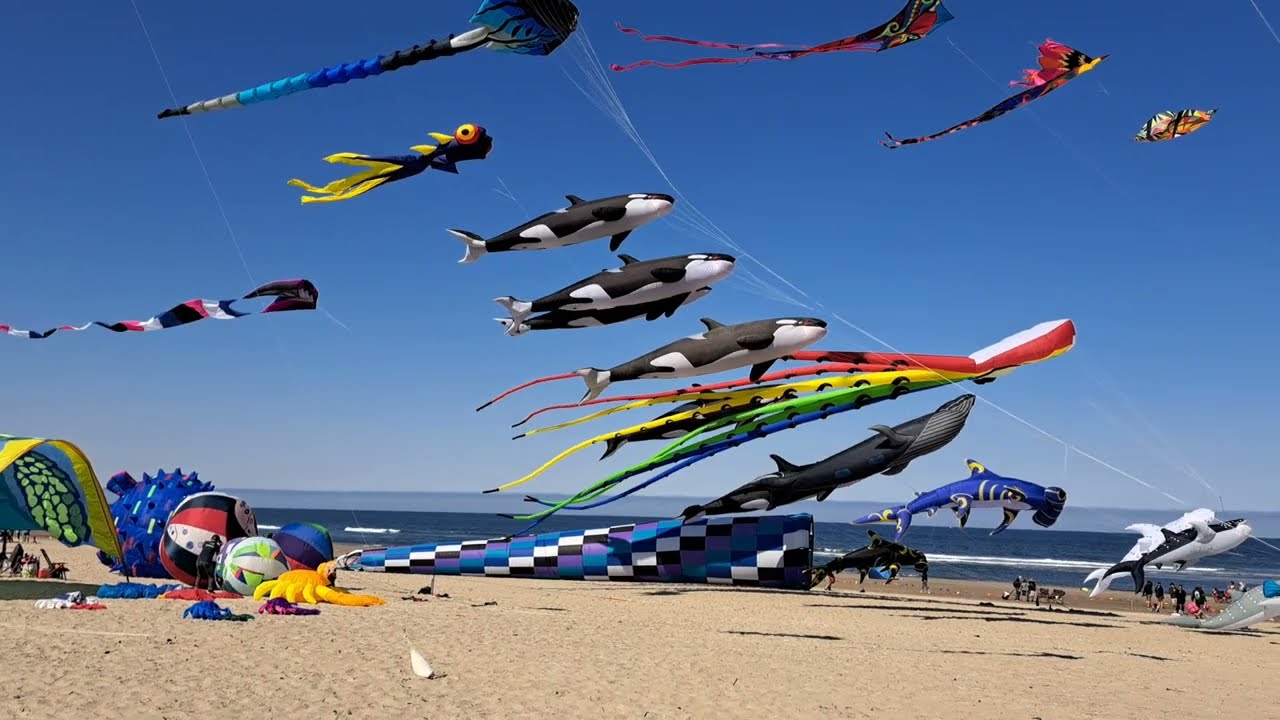The photograph captures a vibrant kite festival set on a picturesque beach. The lower half of the image shows the sandy beach scattered with several tents in the bottom left corner, transitioning to the ocean, and then rising into a vast expanse of blue sky that occupies the top 75% of the frame. The sky is filled with approximately 15 kites soaring at various heights, all generally facing to the right. These kites are diverse in shape and vivid in color, depicting sea creatures such as orca whales, sharks, jellyfish, and a rainbow-colored octopus, alongside other designs like butterflies and tubular windsocks. Four black and white killer whale kites are especially prominent, alongside a hammerhead shark and a monarch butterfly. Though few people are visible due to the photograph's angle, the scene is bright and lively, showcasing an array of black, red, white, and blue kites, including some grounded like a yellow crab. The overall atmosphere is cheerful and colorful, perfectly capturing the essence of the festival.